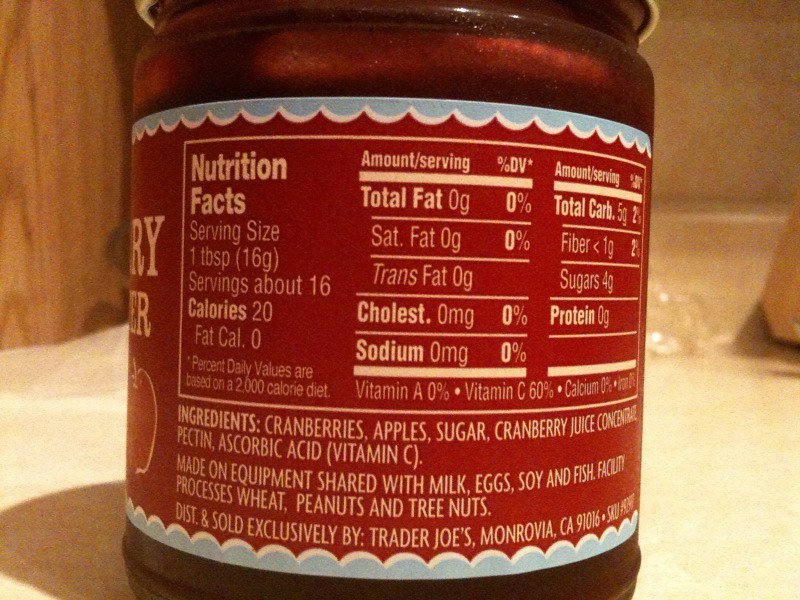The image is a low-resolution, poorly taken color photograph of a cylindrical glass jar with a white cap, placed on a white table. The contents inside the jar are a reddish-brown substance, suggesting it might be a cranberry product, such as cranberry jam. Most of the jar's label is visible, though it's primarily showing the back, which displays a nutritional facts table and ingredients list. The label features a design with light blue, cloud-shaped borders at the top and bottom, and a red middle section with white writing. Key ingredients listed are cranberries, apples, sugar, cranberry juice concentrate, pectin, and ascorbic acid (vitamin C). The product is distributed by Trader Joe's, based in California. Additionally, the label showcases the serving size, calories, and nutritional percentages, including 60% of daily vitamin C. A small red berry image with white borders is depicted on the bottom left of the sticker.